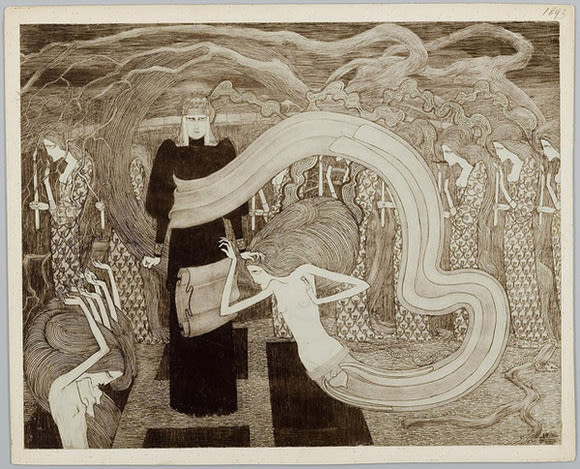This is a detailed black and white drawing, with hints of aging beige tones, possibly dating back to 1893. Framed with a white border, at the center stands a androgynous figure in black robes, possibly a priest, exuding a stern, intense gaze. Their right hand seems to be pushing down the head of another feminine-presenting figure whose body extends into a long, ribbon-like wavy form that spirals around the central figure. This spectral figure has flowing hair and a naked upper torso, accentuating an eerie, ethereal presence.

On the left side of the drawing, at the bottom, two shirtless women raise their hands as if in worship, their hair flowing in tandem with the spectral elements of the scene. Above them, a woman holding a candle looks away from the central figure. To the right, additional women clothed in strange, patterned dresses, stand with arms raised, some holding candles. These women appear to have smoky, branching elements extending from them, merging with the twisted trees in the background, which enhance the overall eerie and dark ambiance of the illustration. Tombstones are scattered around the central figure, suggesting a graveyard setting as an ominous backdrop.